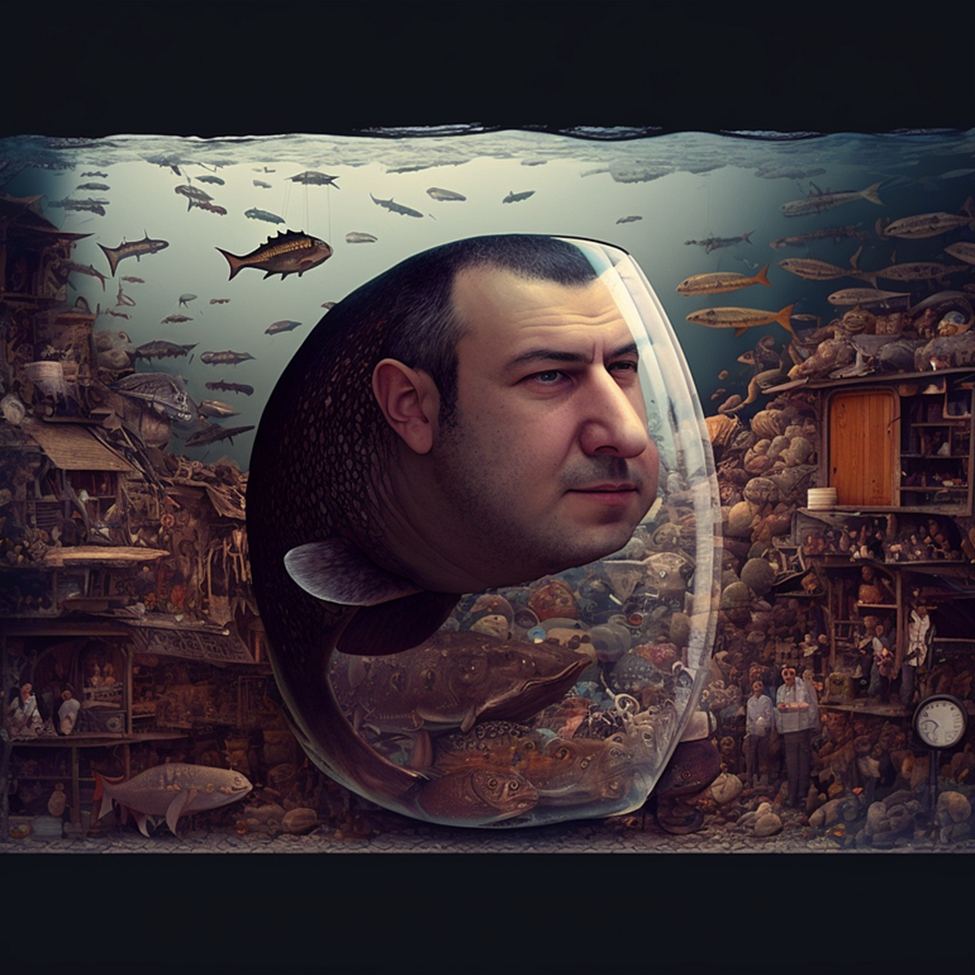The captivating image presents a surreal, underwater scene reminiscent of a magical, aquatic dream. Dominating the center of the image is what appears to be a large, glass-like bubble or bowl, occupying roughly a quarter of the entire frame. Within this bubble, a distorted yet striking visage of a white male with very short hair and a light mustache gazes towards the right. His face intriguingly transitions into the body of a fish, complete with small fins on his neck, rendering him part human, part aquatic creature. The backdrop within the bubble includes other fish and what seems to be a turtle shell.

Encircling the bubble, the underwater environment is teeming with life and activity. The deep blue water fills the frame from edge to edge, with a faint black bar at the top indicating the water's surface. Shelving units and pottery add an enigmatic touch, hinting at an underwater cityscape. Various fish of different shapes and sizes swim across the scene, with many thin, beige-colored fish on the right swimming leftward. A larger, spiky-finned fish is particularly prominent on the left.

Additionally, at the bottom of the image, one can see people standing along what appears to be the ocean floor, contributing to the image's overall ethereal quality. The clear, well-lit image offers a fantastical blend of marine life and human elements, capturing a magical, almost otherworldly underwater world.